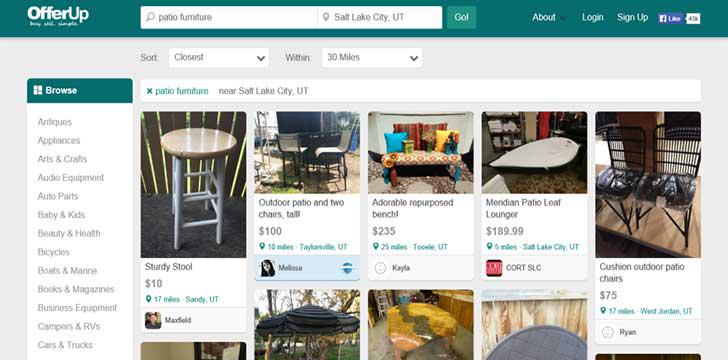This screenshot from the OfferUp website features a user interface designed for searching and browsing items for sale. At the top of the image, there is a prominent green banner. In the left corner of the banner, "OfferUp" is displayed in white text. Adjacent to this is a search bar with black text inside that reads, "patio furniture in Salt Lake City, Utah." 

Located on the right side of the green banner, there are several buttons labeled "About," "Log In," "Sign Up," and a Facebook "Like" button.

Beneath the banner, the webpage background is a subtle grayish-white tone. On the left side of the page, there is a vertical navigation column titled "Browse." This column has an extensive list of category buttons including: Antiques, Appliances, Arts and Crafts, Audio Equipment, Audio Parts, Baby and Kids, Beauty and Health, Bicycles, Boats and Marine, Books and Magazines, Business Equipment, Campers and RVs, and Cars and Trucks.

The main section of the page displays various colorful photographs of patio furniture listings. These items include:
- A stool priced at $10.
- An outdoor patio set with two tall chairs priced at $100.
- An adorable repurposed bench listed for $235.
- A Meridian patio leaf lounger priced at $189.99.
- Cushion outdoor patio chairs available for $75.
Additionally, there is an image of a patio umbrella amongst the listings. 

This detailed screenshot illustrates the functionalities and aesthetic layout of the OfferUp website, focusing on the search results for patio furniture in Salt Lake City, Utah.